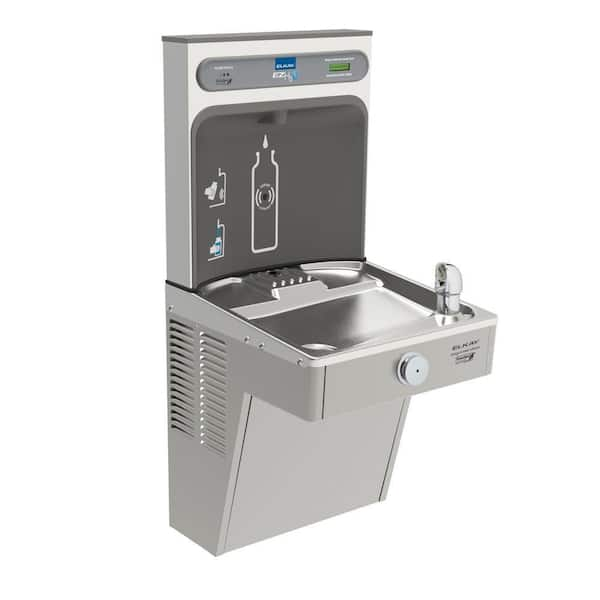This image displays a modern, stainless-steel wall-mounted water fountain against a plain white background. The sleek unit, commonly found in public places like hospitals, universities, and stores in the United States, features a traditional spout for drinking water along with a prominent secondary dispenser designed for filling water bottles. This bottle-filling station includes a top-loading outlet recessed in a dark gray alcove, complete with a diagram and arrows illustrating how to properly position the bottle. The water fountain has a digital readout along the top and ventilation openings on the bottom left-hand side. It also has a push button for water flow. Despite the sharp and shiny appearance of the stainless steel, making the unit look brand new, the manufacturer's logo below the drinking spout remains unreadable due to its small size.